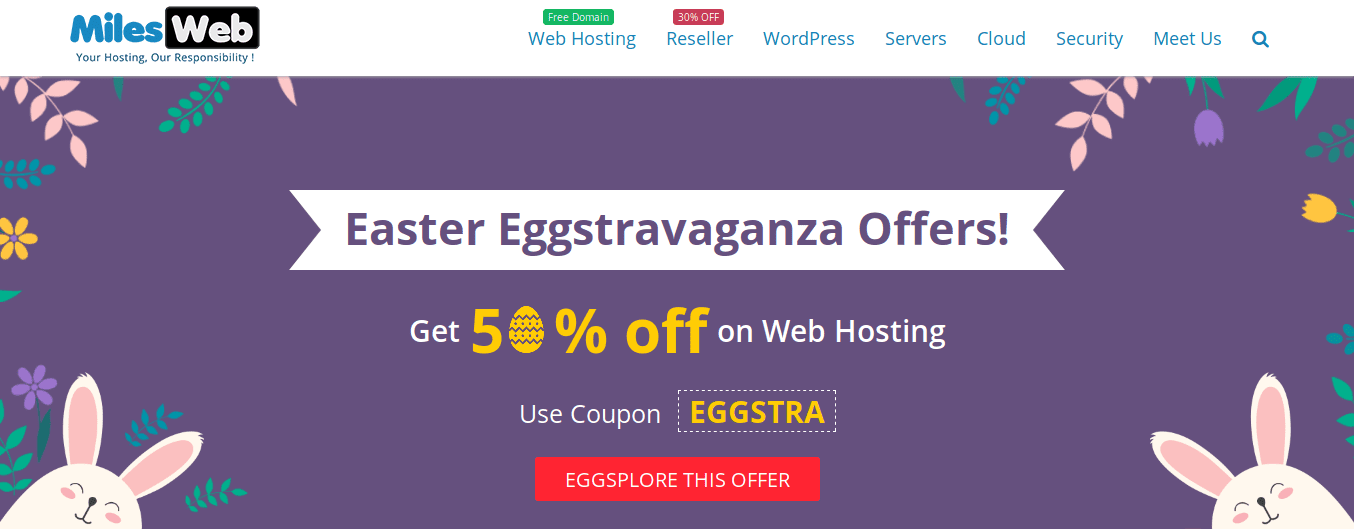**Image Description:**

The image appears to be a promotional advertisement for a web hosting service, designed with a festive Easter theme.

**Header:**
- At the top right corner, the word "Miles" is prominently displayed in bold blue font.
- Adjacent is a black rectangle with "Web" written in white font.
- Below this, a tagline states, "Your housing, our responsibility."

**Top Center:**
- A green rectangle with white font reads, "Free Domain."
- Next to it, a red rectangle with white font offers "30% Off."
- Below "Free Domain," the phrase "Web Hosting" is displayed.
- Under "30% Off," the term "Reseller" is written.

**Right Section:**
- Key terms are listed: "WordPress," "Servers," "Cloud Security," "Meet Us."
- A magnifying glass icon indicates a search function.

**Main Body:**
- The background is a vibrant purple with various colorful clip-art images: purple leaves, pink leaves, orange flowers, and tulips in shades of orange and purple.
- At the very bottom corners, drawings of bunnies enhance the Easter theme.
- The text "Easter Extravaganza Offers" announces the seasonal promotion.
- Below, it states, "Get 5%" (with a drawing of an egg instead of the number five) "Off on Web Hosting."
- The coupon code is "EGGSTRA" (E-G-G-S-T-R-A).

**Call to Action:**
- A red rectangle invites users to "Explore This Offer" in white font.